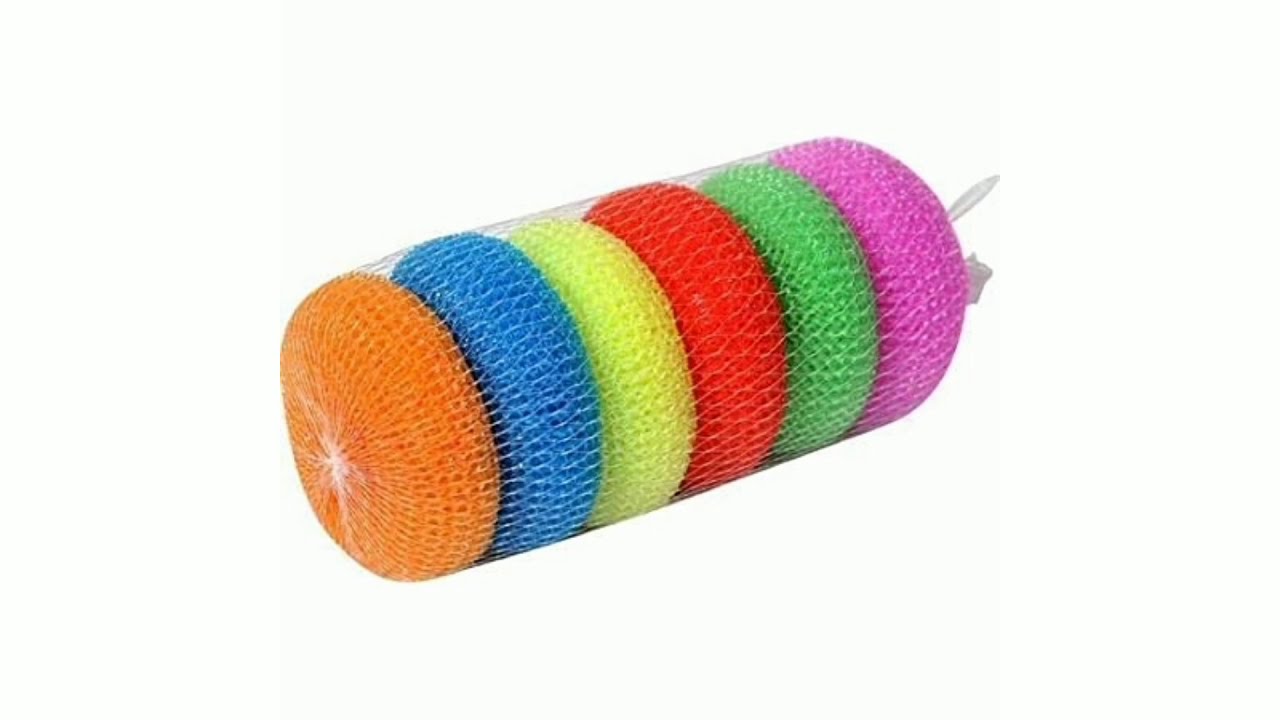The image displays a package of six colorful bath loofahs arranged within a clear white mesh bag. Positioned at a slight 45-degree angle, the bag extends from the lower left to the upper right, resting flat against a spotless white background. The loofahs are orderly stacked, with an orange one at the bottom, followed by blue, yellow, red, and green, and topped with a purple loofah at the peak. The texture of the loofahs suggests they are made from thin, squishy plastic mesh, ideal for scrubbing in the bath. The top tie of the mesh bag is visible slightly to the right of the purple loofah, while the bottom section of the bag features a core piece of mesh that provides a clear view of all six vibrant loofahs. The high-quality image is devoid of text or other objects, allowing full focus on the neatly arranged, colorful loofahs in the center.